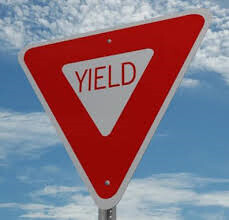A square photograph captures the top portion of a yield sign prominently featuring the bold red text "YIELD" against a light backdrop. The sign shows visible JPEG artifacts, indicating a moderate-to-low image quality. Fastened by two central studs and additional studs along its sides, the sign stands out clearly. Behind it, a blue sky dotted with scattered cirrus clouds suggests it is a sunny day, although the sun itself is not visible. The lack of surrounding landmarks such as trees or telephone poles hints that this sign is likely located on a secluded highway. The image includes just a small part of the pole that supports the sign, enhancing the focus on the yield sign itself.